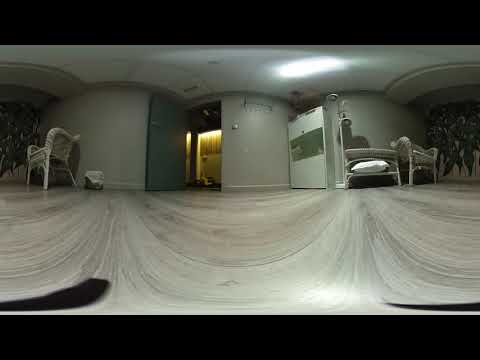The image captures a panoramic view of a room from a low camera angle, which distorts the appearance of the white marble floor with black streaks, making it look wavy. The room's ceiling is composed of white panels with a single long light in the center. The predominantly white and gray walls contribute to a minimalist aesthetic. On the right side of the room, there’s a bare white cabinet with a cut-out section in the middle and a small drawer on top. Adjacent to the cabinet, a table holds a white lamp and appears to store a bag underneath. A white chair faces the camera near the center-right. To the left, a blue door, resting open, leads to an exterior area with a pillar and yellow lighting. There's also a small white trash can with a black bottom and another white chair facing left. The left wall features patterns or murals in shadow, including an indiscernible black figure design, while the right wall also shows patterns, possibly contributing to the room’s sparse decor along with a wicker chair positioned against it. The overall room feels spacious and open, with a doorway illuminated by warm yellow light, contrasting with the otherwise monochromatic palette.